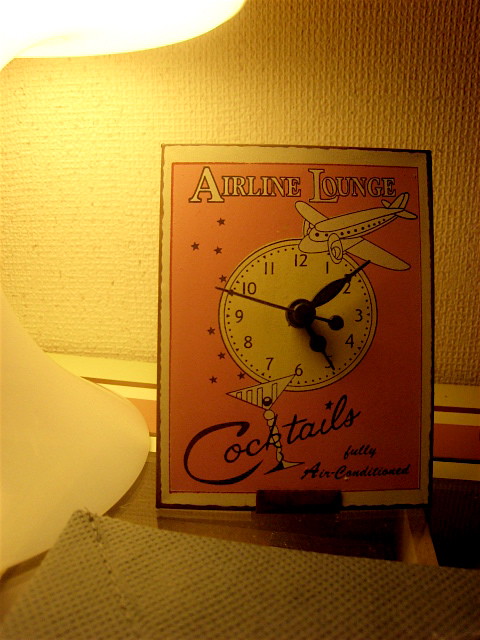This image features a small, vintage-style clock crafted from metal. The clock's top bears the inscription "Airline Lounge," accompanied by an airplane graphic just above the circular clock face. The clock face showcases two main hands alongside a third, smaller hand. The background of the face is a vibrant pink, encased within a white border, and the text is rendered in a combination of black and white fonts. Below the timepiece, the words "Cocktails" and "Fully Air Conditioned" are prominently displayed, with a wine glass icon cleverly integrated into the word "Cocktails." The clock stands upright, supported by a small stand. In the foreground, a cloth, possibly a napkin, is laid out, while the background reveals a textured, wallpaper-covered wall. An unidentifiable object is positioned to the left of the clock, adding an element of intrigue to the setting.